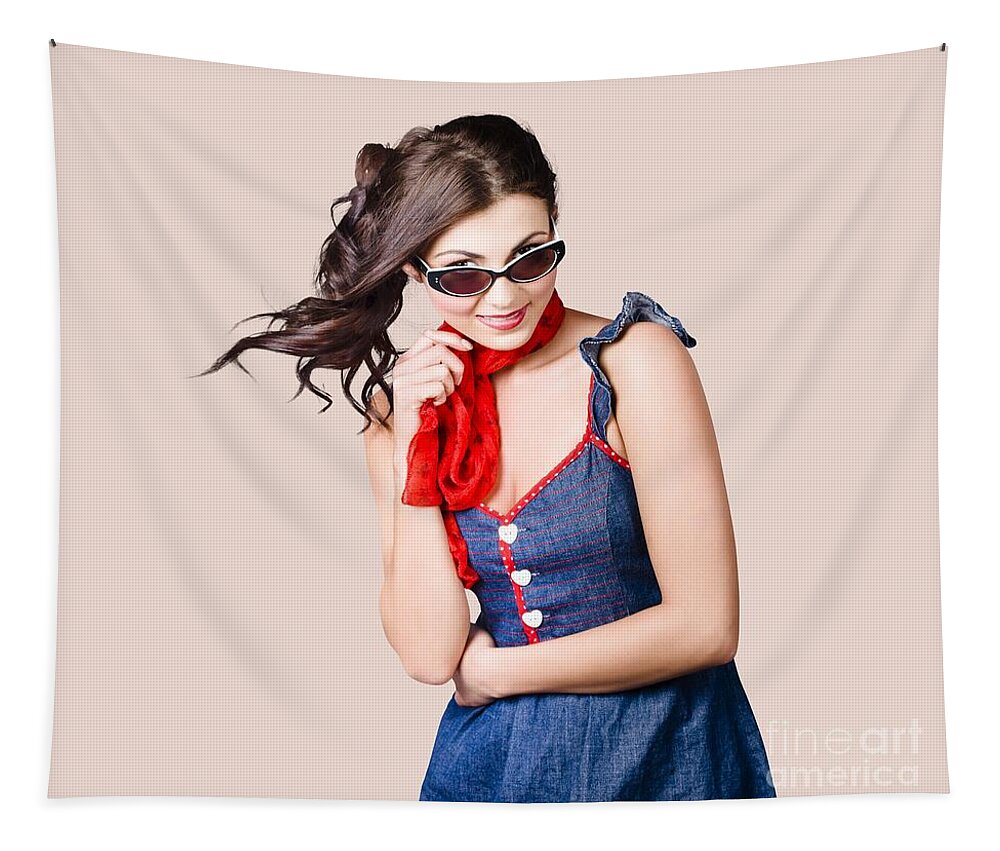The image depicts a woman wearing a blue denim-style dress with spaghetti straps covered in denim material. The dress features a striking red trim around the top and running down the front, complemented by three prominent heart-shaped buttons that add a whimsical touch. She accessorizes with a cherry red, silky scarf, which she holds elegantly with her right hand, while her left hand rests around her waist. Her long, dark brown hair cascades to her right side, appearing windswept and slightly messy. She sports a pair of vintage, pointy sunglasses and is gazing towards the camera, peering just over the top of her glasses. The scene is rendered on a tan or beige fabric backdrop, possibly a blanket, which is tacked to the wall. The bottom right corner of the image features a small watermark reading, "Fine Art America."